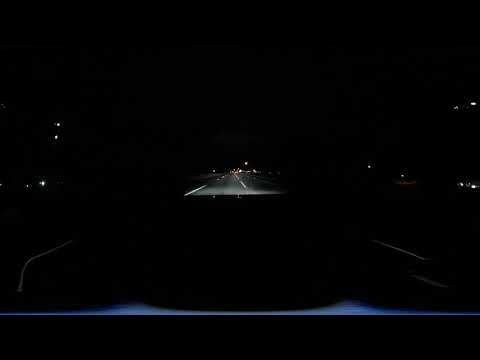The image is a photographic, nighttime scene captured from the perspective of someone driving down a dark highway. The setting is outdoors, and the photo has a dashcam feel, possibly a screenshot of a video. The road is a grey, two-lane highway with a center stripe, illuminated by the car's headlights. The foreground shows a puzzling curved blue line that could be the hood, stretching horizontally with light blue glow at two points left and right of the center. 

In the distance, small yellow light sources are scattered, suggesting reflectors or faint streetlights, with about six on the right side and two or three on the left side of the road. These lights seem reflective rather than illuminating. Additionally, there might be another vehicle's headlights in the opposing lane, hinting at a sparse traffic presence. 

The overall background is pitch black, creating a stark contrast with the limited, visible elements. This gives the image an eerie, solitary feel, as the driver's headlights cut through the darkness, highlighting the road and its markings amid mostly obscured surroundings.